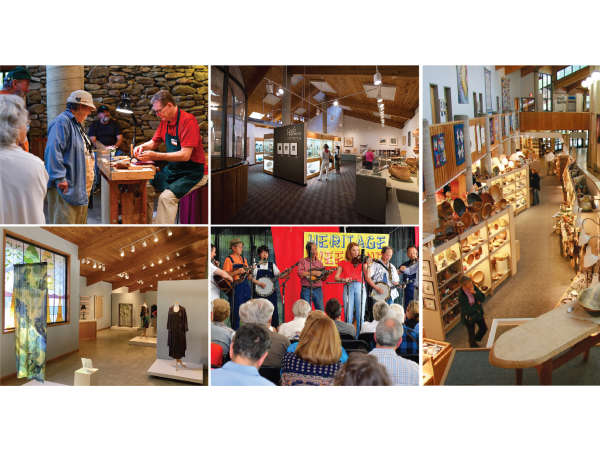The collage features five distinct images, intricately capturing a vibrant scene within a museum or craft fair setting. In the top left corner, a man in a red shirt and apron is engaged in a creative endeavor, drawing the attention of an elderly lady in a hat who seems interested in his work. The top center image reveals a spacious room with wooden ceilings and several people scattered within, highlighting a well-lit and warmly adorned interior. Adjacent on the top right, a taller vertical image showcases another expansive room filled with wooden craft materials displayed on various shelves, with people closely examining the artistic items. The bottom center image offers a lively glimpse of a stage performance, where several musicians equipped with instruments such as banjos and violins entertain an audience seated before them. Finally, the bottom left image portrays an interior room adorned with mannequins displaying an array of fashion items, underlining the aesthetic continuity of wooden beams and high ceilings in the overall design. This detailed collage collectively portrays a space bustling with artistic creation, display, and performance, encapsulating a rich atmosphere of cultural appreciation and interaction.